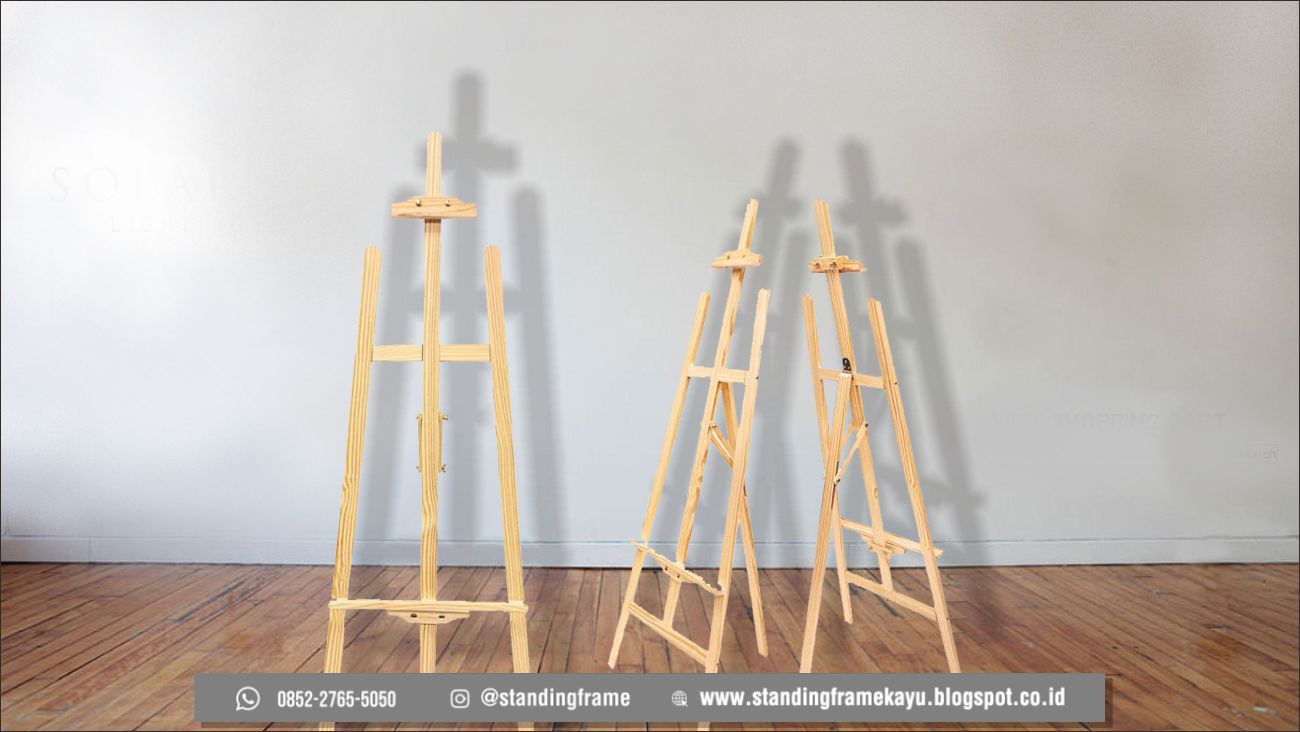This color landscape image, which is difficult to discern as either a real photograph or a digital render due to its quality, features a detailed depiction of three wooden easels positioned on a dark, wood-paneled floor. The floor, occupying the bottom quarter of the image, showcases a variety of shades with light, dark, and black patches highlighting the wood grain, and the floor panels run from front to back. Central to the image are the three light beech pine easels, arranged sporadically. The closest easel, on the left, faces directly toward the viewer, positioned as if ready to hold a canvas. The two other easels are facing different directions; one points diagonally forward and to the left, while the other faces away. Each easel, designed with two long side legs, a central supporting leg, two back crossbars, and a ledge for holding canvases, casts partial shadows on the floor and a wall behind them.

The backdrop features a wall that transitions from brilliant white on the left to patches of grey and tinges of yellow and brown on the right, indicating signs of aging or dirt. At the top of the image, there is a grey rectangular banner containing social media symbols and text. This banner includes a WhatsApp symbol with a phone number, an Instagram symbol followed by "@StandingFrame," and another symbol that is too blurry to identify, with a website listed as "www.standingframe.blogspot.co.id."

Overall, this image appears to be a product display for wooden easels, complete with social media and contact information.